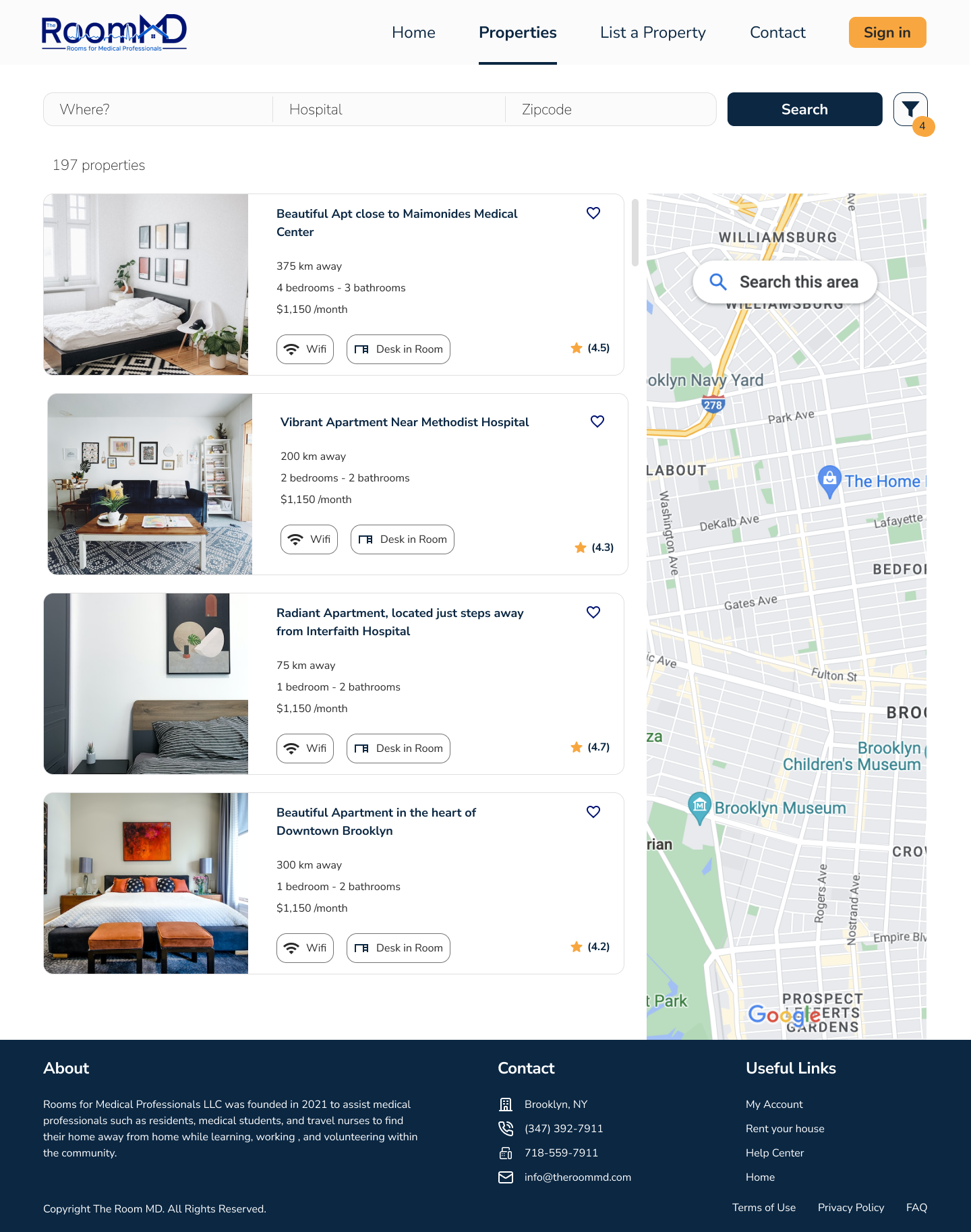The screenshot depicts a section of a website named "RoomMD," which caters to rental properties for medical professionals such as travel nurses, residents, and medical students. The RoomMD logo features blue text with lighter blue accents, with the tagline "rooms for medical professionals" underneath.

The navigation bar at the top of the website has a gray background and includes options such as "Home," "Properties," "List a Property," "Contact," and a "Sign In" button. Below this is a search bar with fields labeled "Where," "Hospital," "Zip Code," and a blue "Search" button along with a filter icon.

Displayed on the page are summaries of the listings available. The webpage indicates a total of 197 properties, with only four shown on this particular screen, and a map of the Williamsburg area in New York displayed to the right of the listings. It is identifiable as New York from the listed locations and directional signage mentioning Brooklyn and Williamsburg.

**Property Listings:**

1. **Beautiful Apartment Close to Maimonides Medical Center**
   - Distance: 375 kilometers away
   - Features: Four bedrooms, three bathrooms, Wi-Fi, desk in the room
   - Price: $1,150 per month
   - Rating: 4.5 stars
   - Image Description: A brightly lit room with a white bed on a black frame, a black-and-white patterned carpet, a small plant in the corner, and colorful frames on the wall.

2. **Vibrant Apartment Near Methodist Hospital**
   - Distance: 200 kilometers away
   - Features: Two bedrooms, two bathrooms, Wi-Fi, desk in the room
   - Price: $1,150 per month
   - Rating: 4.3 stars
   - Image Description: A brightly lit room featuring a bluish couch, a large wooden coffee table with white legs, a patterned rug, and a gallery wall with frames.

3. **Radiant Apartment Located Just Steps Away from Interfaith Hospital**
   - Distance: 75 kilometers away
   - Features: One bedroom, two bathrooms, Wi-Fi, desk in the room
   - Price: $1,150 per month
   - Rating: 4.7 stars
   - Image Description: Mostly a white wall with an off-centered photo showing part of a bed with black-and-white bedding and a wooden headboard, plus a modern wall image.

4. **Beautiful Apartment in the Heart of Downtown Brooklyn**
   - Distance: 300 kilometers away
   - Features: One bedroom, two bathrooms, Wi-Fi, desk in the room
   - Price: $1,150 per month
   - Rating: 4.2 stars
   - Image Description: A spacious, brightly lit room featuring a large bed with orange, black, and white pillows, matching nightstands, a red wall art piece, and bench seats at the foot of the bed.

At the bottom of the screenshot, there are sections for "About," "Contact," and "Useful Links." The "About" section provides information about Rooms for Medical Professionals LLC, which was founded in 2021. It explains the company's mission to help medical professionals find accommodations while working or volunteering in the community. 

**Contact Information:**
- Location: Brooklyn, New York
- Phone: 347-392-7911
- Fax: 718-559-7911
- Email: info@theroommd.com

**Useful Links include:**
- My Account
- Rent Your House
- Help Center
- Home
- Terms of Use
- Privacy Policy
- Frequently Asked Questions

This detailed and structured caption provides a comprehensive description of the website and the information displayed on the page.